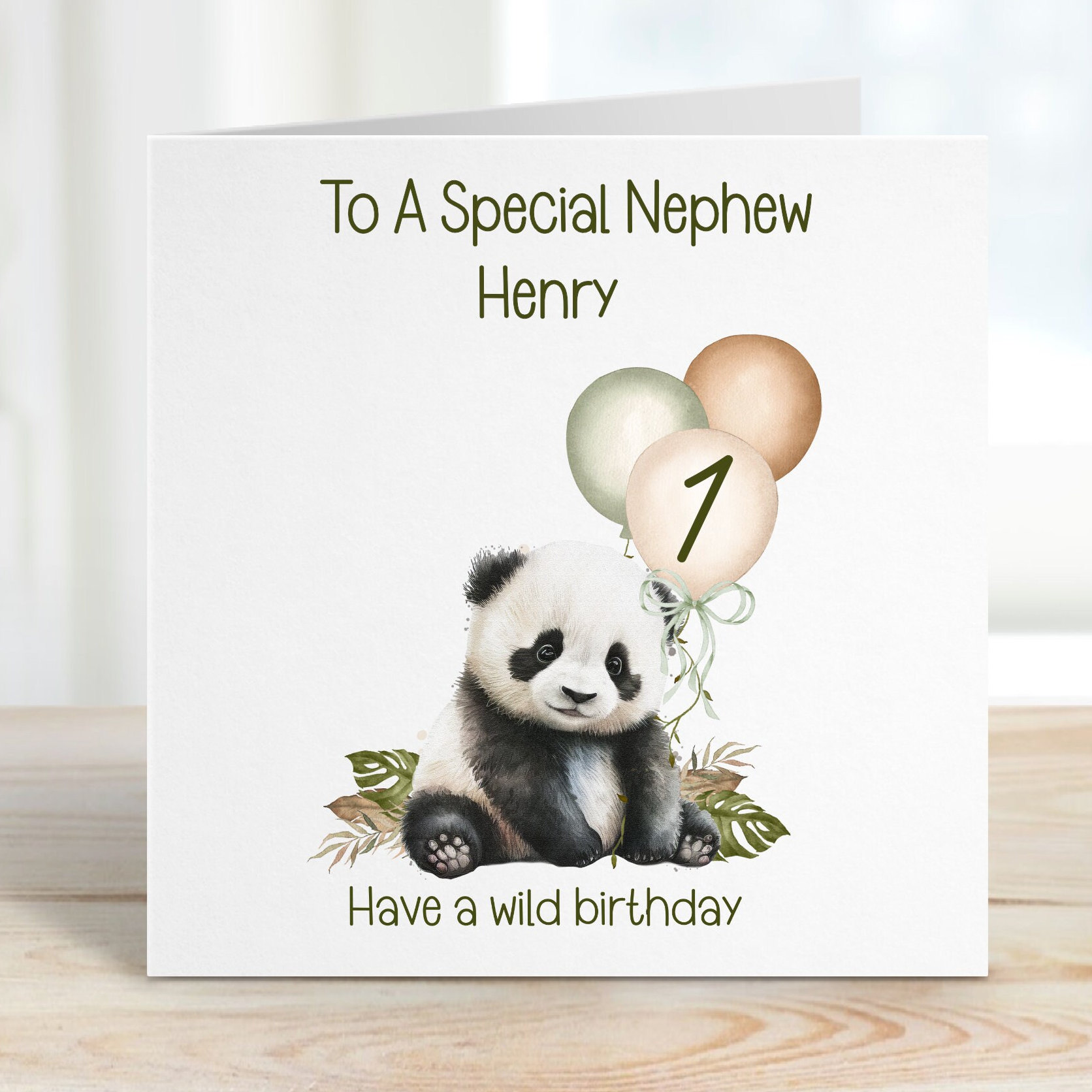This photograph captures an adorable birthday card positioned against a white wall on a light brown wooden floor. The card itself is primarily white and beautifully illustrated with an endearing baby panda, with white fur, brown blotches on the left side of its head and underneath its chin, black ears, arms, feet, and a white belly. The baby panda sits contentedly among an array of leaves—green and brown ones on either side, with a broken brown leaf on its left. Above the panda float three colorful helium balloons: a green balloon, an orangish-brown balloon, and an off-white balloon outlined in brown with the number one on it. Additionally, a green bow accents the right side of the panda. The heartfelt message on the card, in green text at the top, reads, "To a special nephew, Henry," while the bottom text, centered beneath the baby panda, says, "Have a wild birthday!" The overall scene is lit from the right, casting a light shadow behind the card, adding depth and warmth to this charming celebratory greeting.